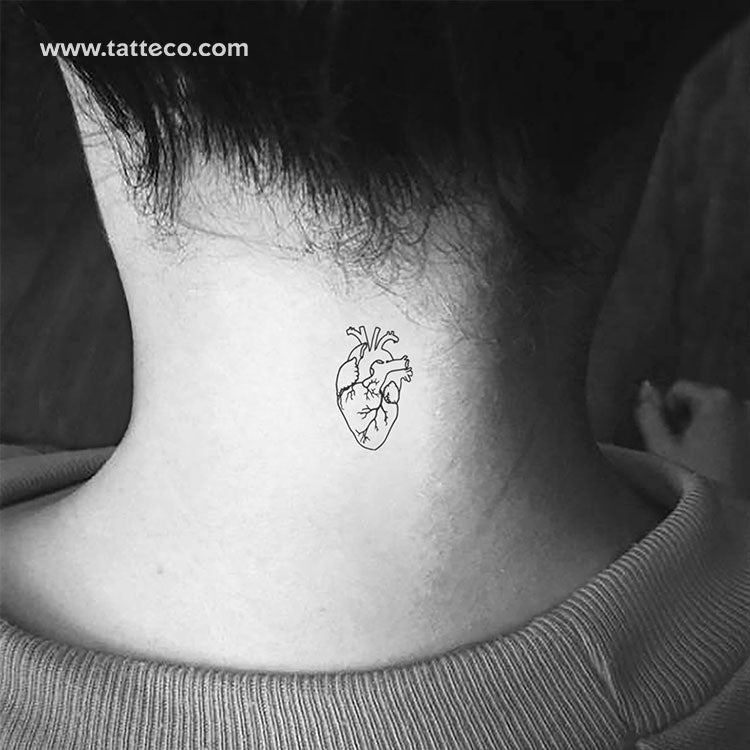This is a detailed black and white photograph focusing on the back of a woman's neck, adorned with a striking tattoo. The woman has dark black hair pulled up above her head, revealing her fair olive skin. Central to the image is a realistic black and white tattoo of a human heart, complete with detailed arteries, veins, and vents. She is wearing a sweater with a laced neckline, and only a few strands of her hair are visible. The background includes a dark floor and an out-of-focus woman’s hand on the right side. In the upper left-hand corner of the image, the URL www.tatteco.com is prominently displayed in gray or white letters against the black background, indicating the likely source or context of the photograph.